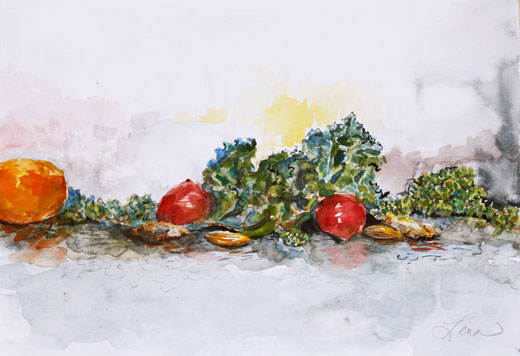This detailed watercolor painting, signed by the artist 'Lena' in cursive at the bottom right corner, predominantly features a still life arrangement with a variety of natural elements. The background is a light grayish-white with smudges of brown, yellow, and some hints of light blue, giving it a marbled appearance. Central to the composition are lush green leaves, which could be kale or lettuce, with variations in shade from dark to light green. Among the leaves, there are two red elements, possibly radishes or tomatoes, characterized by their vibrant color and white streaks. Scattered around these vegetables are oval-shaped brown nuts, potentially almonds, adding texture to the scene. To the left, partially cut off at the edge, is a larger orange object that resembles an orange or possibly a pumpkin, although it lacks a stem. Smaller green leaves are also painted on the right side, completing the intricate arrangement of this still life.